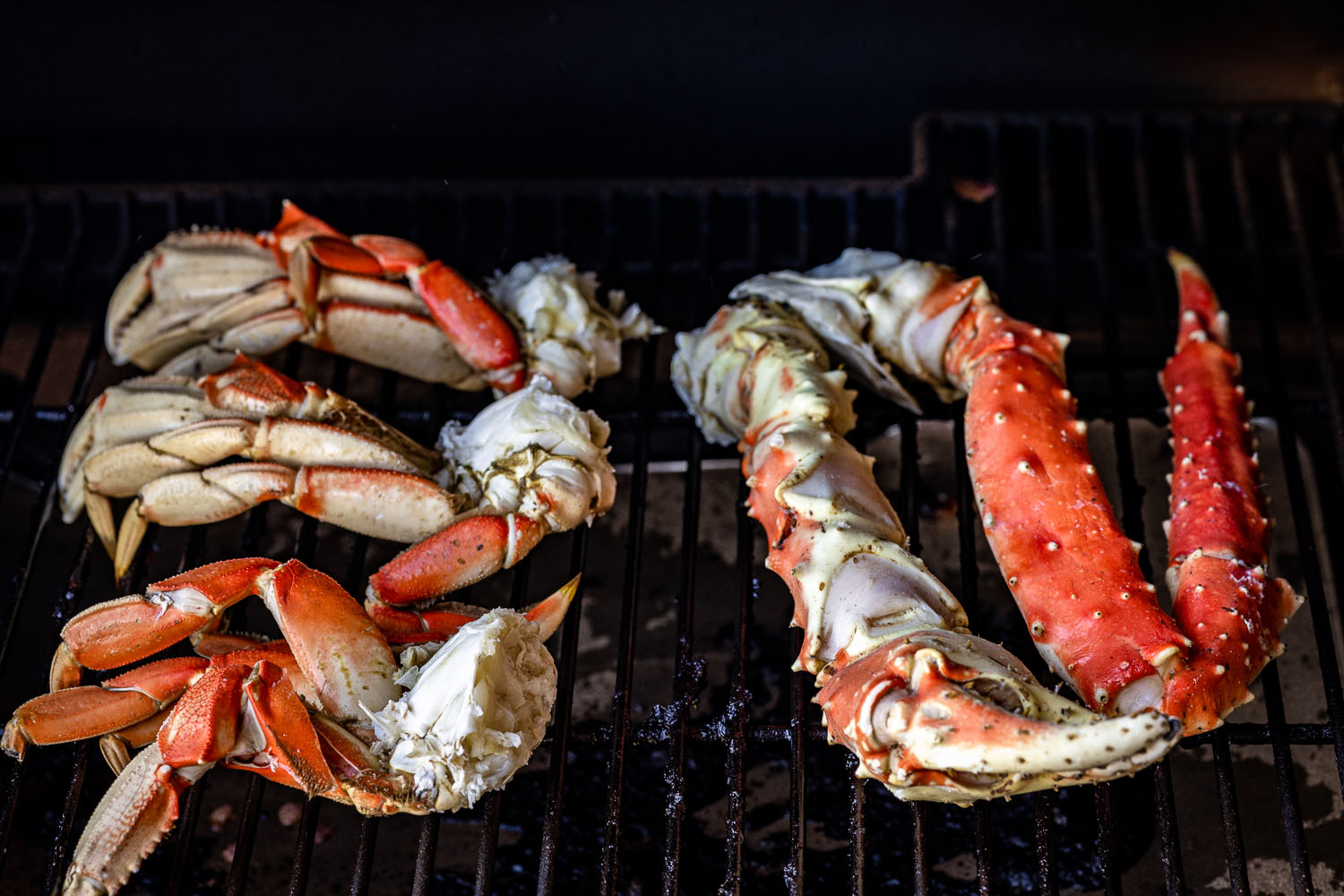This detailed close-up photograph showcases a horizontal grill laden with crab claws and legs in various stages of roasting. The setting, likely indoors, features a dark, nearly black background that accentuates the contrasting vivid colors of the crab. To the left, there are three sets of red, white, and brownish crab claws, appearing to be cut in half and partially cooked, evidenced by their changing hues. On the right, two large king crab legs, one exhibiting a deep reddish-orange tone indicating it’s fully cooked, are meticulously arranged on the grill. Below the grill’s black grating, the charcoal is visible, adding to the bird’s-eye view of this sumptuous scene, with no flames or smoke present.